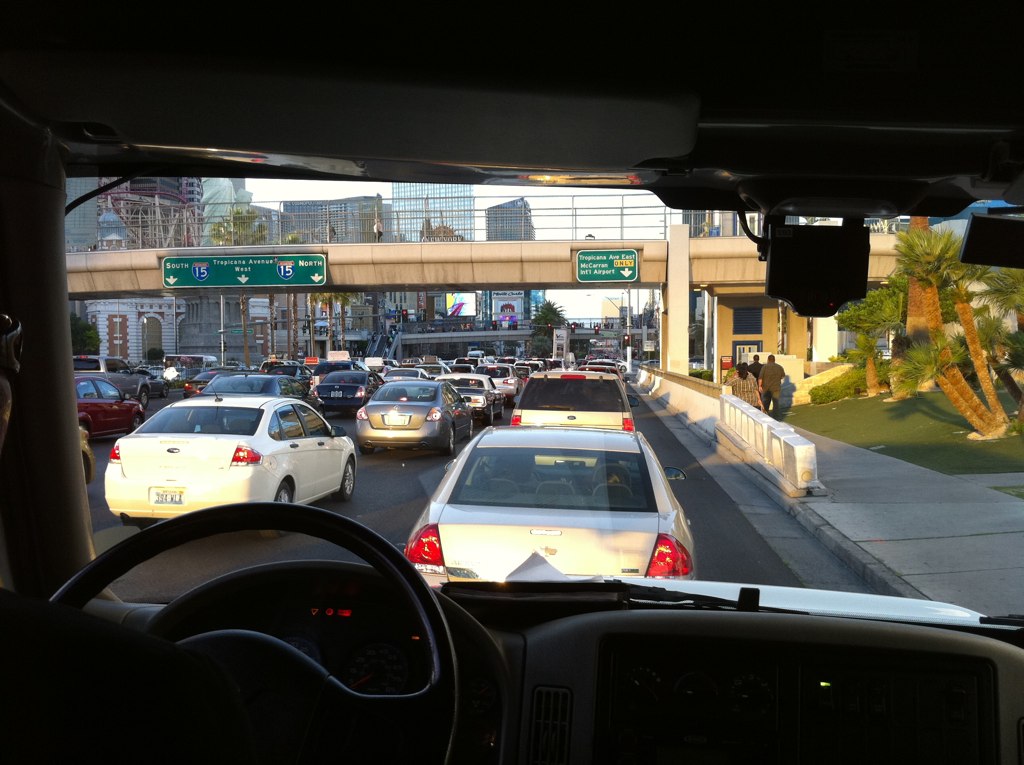The image captures a detailed view of a traffic jam observed from inside a vehicle, likely a truck or van, given the elevated perspective, which allows a clear sightline over the rooftops of the other cars gridlocked on the freeway. The photo is taken from behind the dark silhouette of a steering wheel and a dimly lit dashboard. Through the windshield, several lanes of vehicles are seen idling, stretching out towards an overpass in the distance. The overpass is adorned with multiple green road signs, providing directions for northbound and southbound traffic, as well as listing locations such as Tropicana Avenue East and West, and McCarran International Airport, suggesting that this scene could be in Las Vegas. To the right, a sidewalk accompanies the street, bustling with pedestrians, and small palm trees can be seen adding to the urban atmosphere beneath the skyscrapers that loom on either side of the freeway.